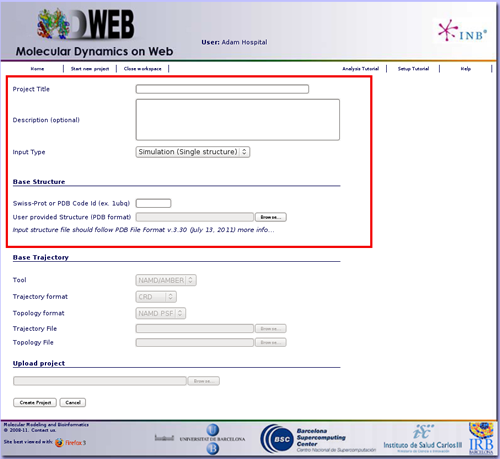Image caption: 

The image depicts a user interface for a web-based molecular dynamics tool named "D-Web" utilized by user Adam at a hospital. At the top of the interface, it prominently displays the label "D-Web Molecular Dynamics" followed by "user Adam hospital." To the right, the interface contains the labels "INB" and a navigation menu with options including "Home," "Start Your Project," and additional, unspecified options due to blurriness.

A red rectangular box is drawn around a section indicating "Project (something)" suggesting it's an important focal area. Below this highlighted section, there's text stating "Description (Optional)," followed by multiple input options for simulation types: "Single Structure," "Basic Structure," and "User Provided Structure."

Further down, although blurry, the image mentions a "Base Trajectory Tool" that supports "MD AMBER Trajectory Format" and "CPD Topology Format," hinting at specialized formats for trajectory and topology handling within the molecular dynamics simulations. The rest of the image is unclear and provides indistinct text.